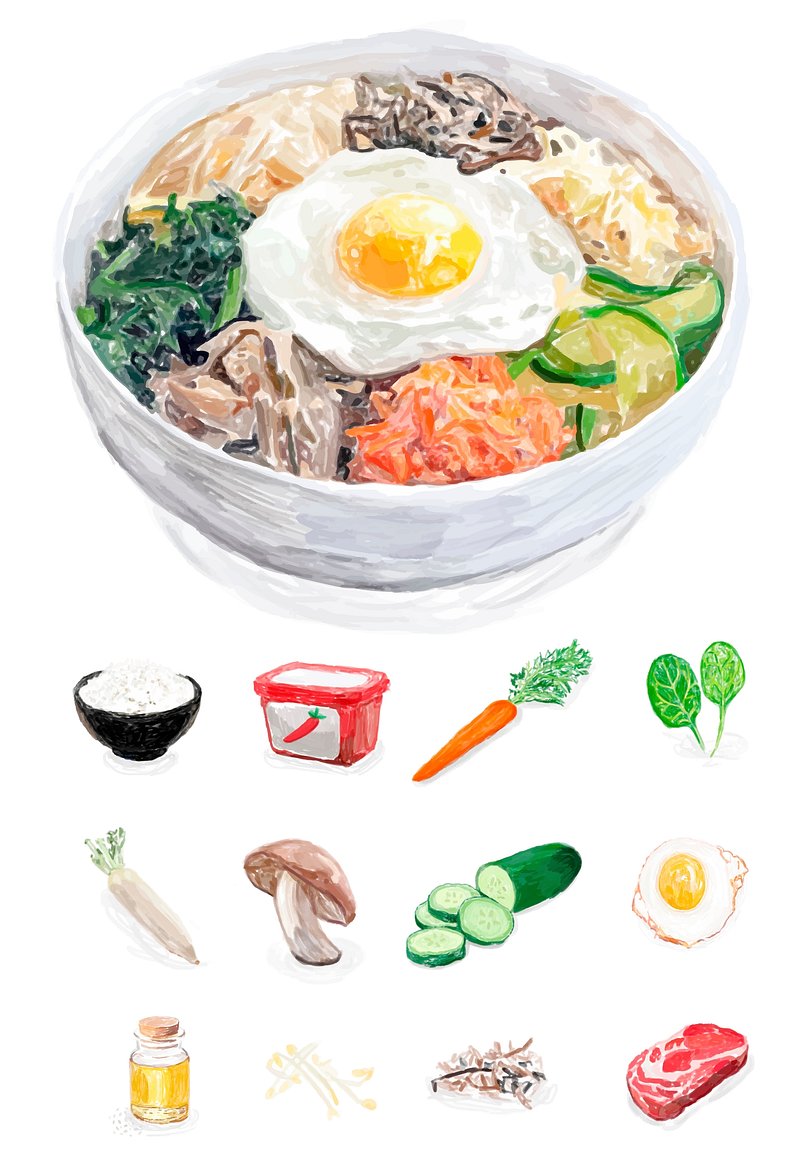This image depicts an acrylic painting of a bowl of mixed food items, prominently featuring a sunny-side-up egg in the center, its bright yellow yolk standing out against the whites. The bowl, located at the top of the image and whitish in color, contains an array of ingredients arranged in a circle. The visible contents include sliced cucumbers, what looks like crushed salmon, and other assorted vegetables and meats, slightly blurred due to the painting style.

Beneath the bowl, there are three rows and four columns showcasing individual food items, possibly indicative of the ingredients in the bowl. In the top row, from left to right, there's a black bowl with white cottage cheese, a red container, a full carrot, and two leaves of mint. The second row includes a mushroom, cut-up cucumbers, a sunny-side-up egg, and a white stalk with a yellow head resembling a type of vegetable. The bottom row displays a tiny jar of honey or oil, some alfalfa sprouts, a piece of steak, and a brown item possibly representing noodles or seasoned food. Each component is distinctly illustrated, although the entire composition maintains a slightly impressionistic quality.